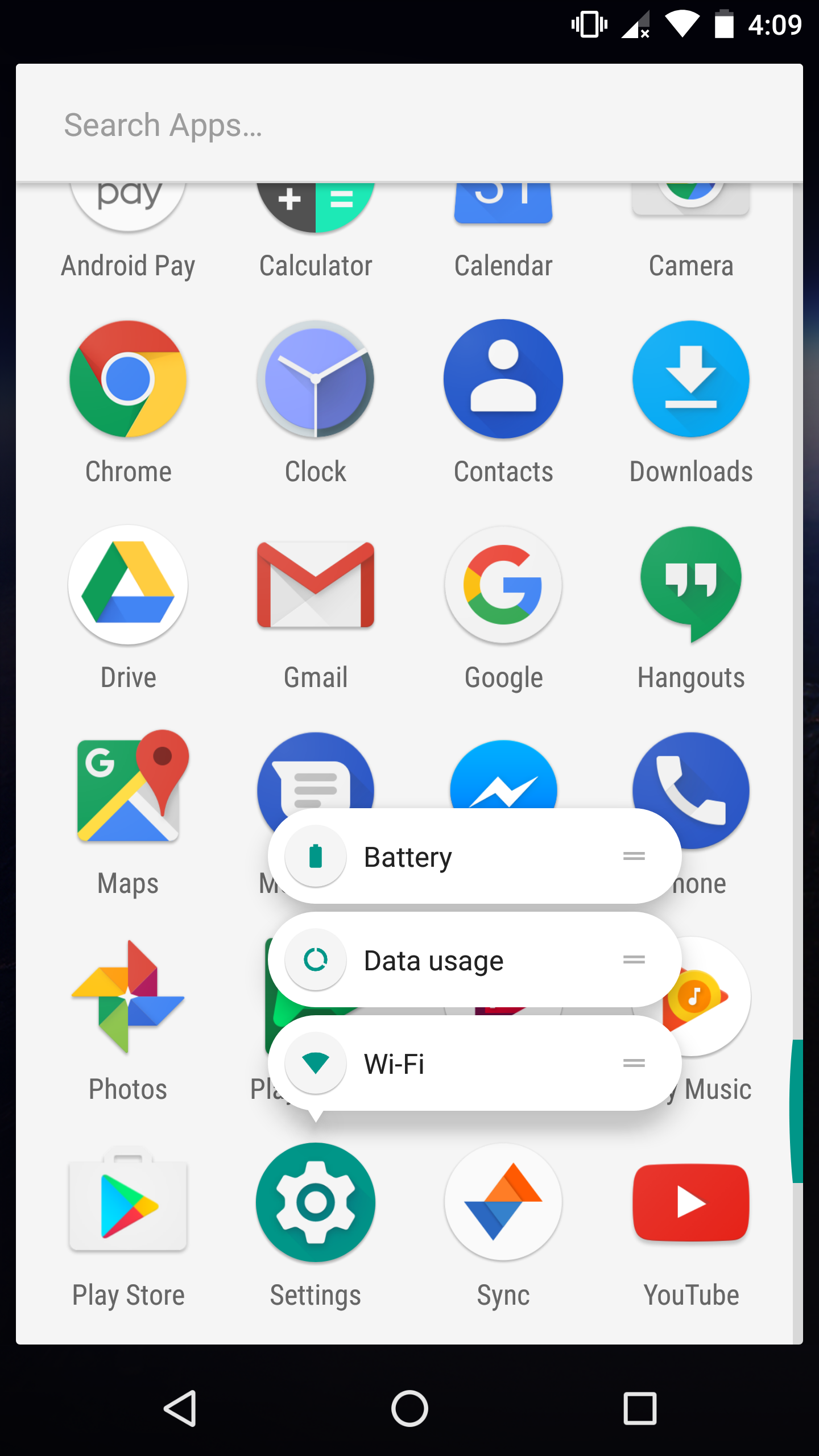A detailed screenshot of an Android phone's app drawer. The captured screen, timestamped at 4:09, shows a nearly full battery level of 98-99%. The top section of the screen features a white background with a black border, housing a prominent search box that reads "Search apps."

Just below the search box, various app icons are displayed, listing the installed applications on the device. Dominant among them are Google's suite of apps, including Android Pay, Google Chrome, Google Drive, Google Maps, Google Photos, Google Play Store, YouTube, Google Music, Phone, Google Hangouts, Google Search, Google Contacts, Gmail, and Google Messages.

At the bottom of the screen, the settings button is highlighted, indicating a long-press action. This action has triggered a context menu with options related to Wi-Fi, data usage, and battery. Each option is styled like a word bubble, and to the right, there is an additional menu option for accessing these settings. The screenshot effectively captures the organized and comprehensive nature of the phone's app drawer and provides contextual details about the available settings and app functionalities.